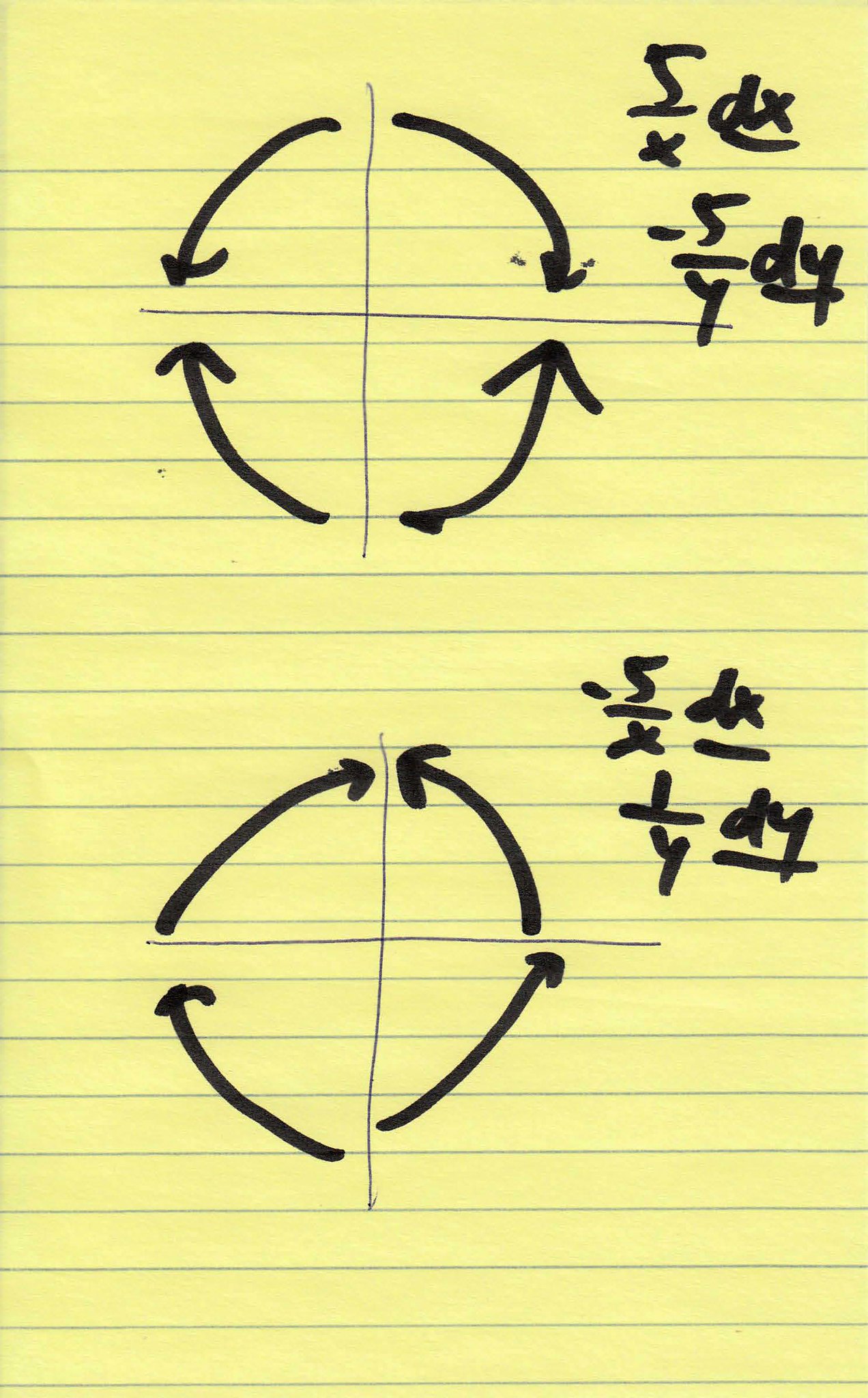This image depicts a yellow legal pad, specifically the smaller 5x7 inch variant, characterized by its distinctive blue horizontal lines. Centered on the top half of the page is a hand-drawn cross, accompanied by four curved arrows arranged to form a circular motion around the cross. The arrows originating from the bottom curve upwards, pointing towards the horizontal segment of the cross, while the arrows from the top curve downwards, aligning with the bottom arrows. Above this diagram, a mathematical expression is written: "5/x dx - 5y dy". Mirroring this diagram on the lower portion of the paper is another cross with the same circular arrow formation, but annotated with a different equation: "5x dx 1/y dy". The notations appear to be mathematical in nature, although their specific meaning remains unclear from the context provided.